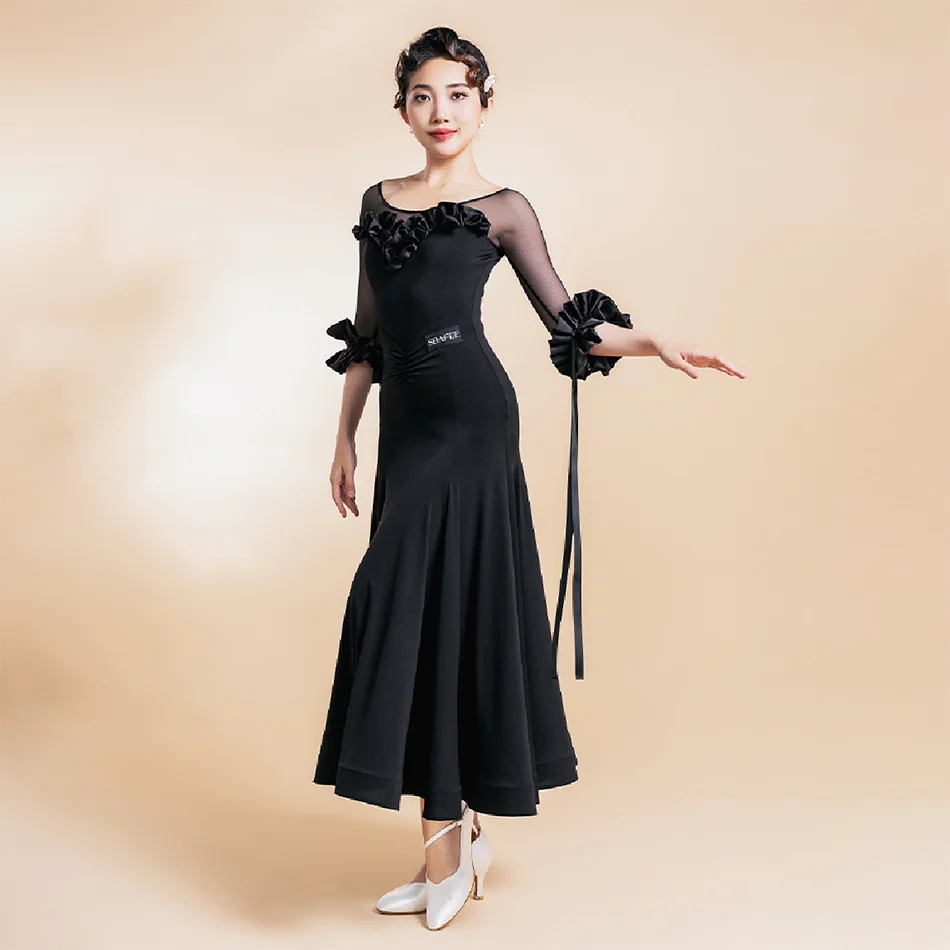This professionally shot image features an Asian woman, possibly of Japanese descent, posed against a cloudy, tannish backdrop. She has striking short, black hair styled in a vintage, 1920s-inspired fashion with a lighter brown curl falling elegantly in front. Her hair is further adorned with barrettes that pull it back neatly. The woman's complexion appears digitally altered, giving her skin a smooth, almost blurred, and flawless appearance. She has a slight, closed-mouth smile and wears a reddish coral shade of lipstick that complements her poised demeanor.

Her attire is a long, black dress extending down to her ankles, characterized by its flowing A-line skirt. The dress has a ruffled bodice forming a V-shape across her chest, and transitions into sheer mesh sleeves adorned with black ruffles and hanging ribbons. One of these ribbons is tied into a bow on her right arm. The sleeves, which stop just below the elbows, feature satin or silk cuffs that add to the dress's elegance. Completing her outfit, she dons low-heeled, white pointy-toed shoes, adding a contrasting touch amid the black ensemble.